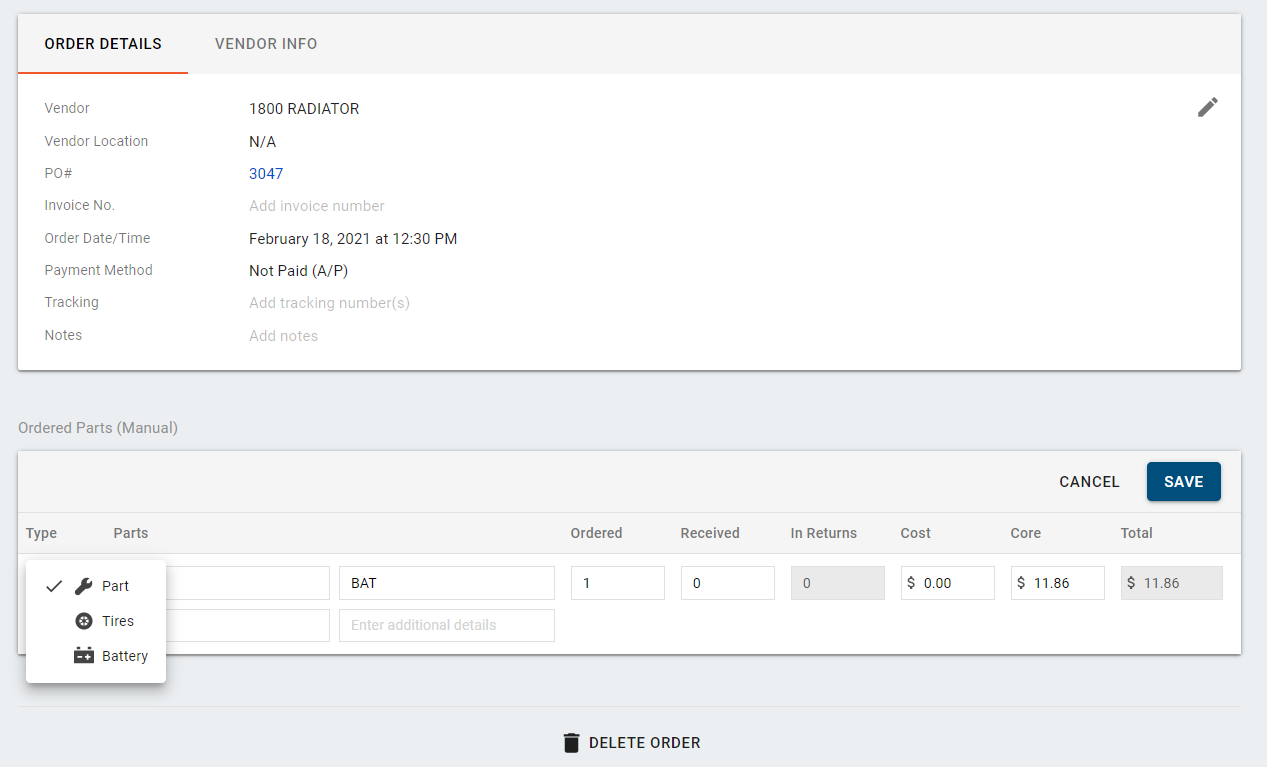Order Details Page Description:

The order details page prominently features information regarding a vendor and a specific purchase order. At the top, the vendor is listed as "1800 Radiator," but the vendor location is marked as "N/A," indicating it's not operable. A clickable P.O. number (3047 in blue) provides access to more information.

Below the P.O. number, there is an "Invoice No" field accompanied by a prompt to add the invoice number. The order date and time are specified as February 18th, 2021, at 12:30 PM. The payment status is noted as "Not Paid," and tracking information is currently unavailable, with options to add tracking numbers and notes.

To the right of this information is a pencil icon, indicating that the details can be edited. Below this, there is a section labeled "Order Parts (Manual)." The type chosen is marked with a checkmark next to "Part," accompanied by a wrench icon. Options for "Tires" and "Battery" are also available for selection.

The parts column is currently blank. To the right, details show "BAT" under the "Back" column, with one item ordered, zero received, and zero returned, which is grayed out. The cost listed is $0, with a core charge of $11.86, making the total $11.86, also grayed out.

The part in question is a radiator component, ordered on February 18th at a cost of $11.86. The background of the page is predominantly white, with gray tabs. The "Save" button stands out as the only colored element, located at the bottom of the page.